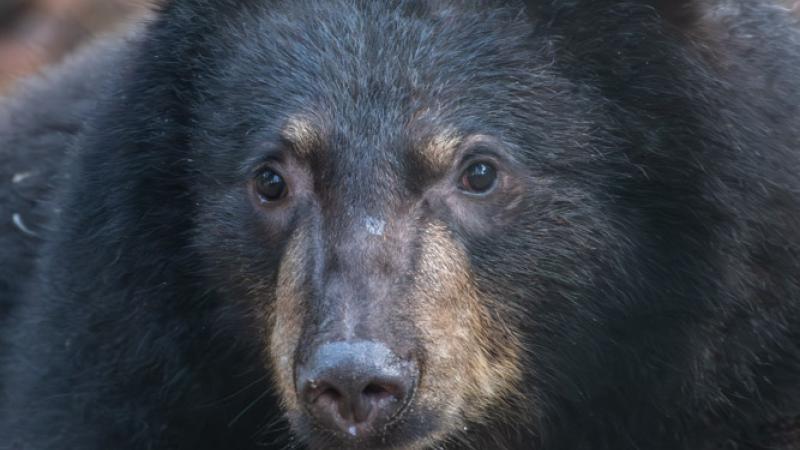This captivating close-up photograph, taken in landscape format, intimately portrays the face of a bear. The bear's striking black fur contrasts with its expressive dark brown eyes and glossy black nose. Notably, patches of light brown fur accentuate its features above the eyes and around the nose and mouth, adding depth and character to its intense gaze. The bear is positioned squarely facing the camera, asserting its presence within the frame. The backdrop is artfully blurred, with a light brown hue peeking through in the upper left-hand corner, subtly hinting at the bear's natural habitat. The composition primarily focuses on the bear's facial details, offering a powerful and endearing glimpse into the world of this majestic creature.